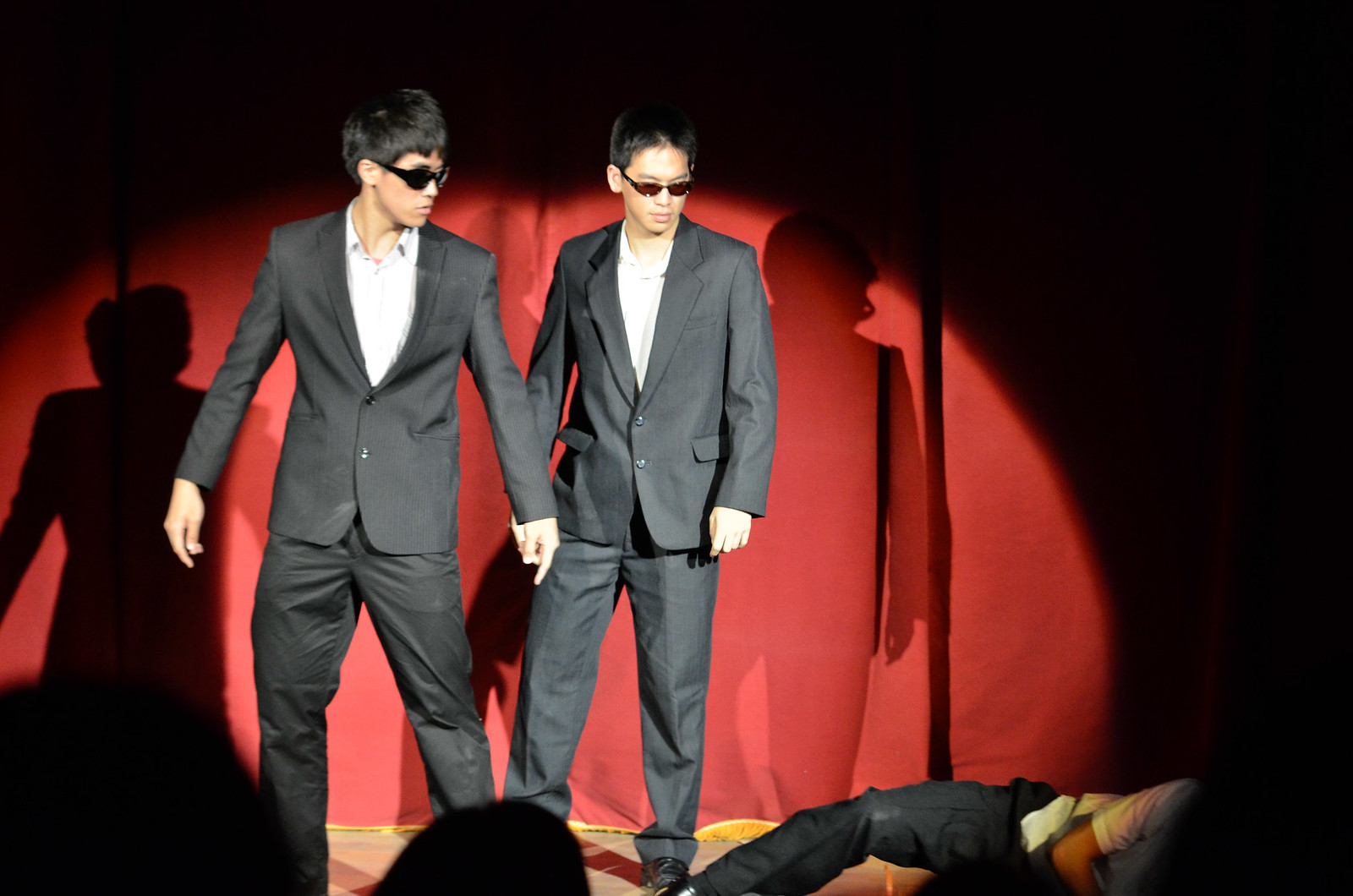In this photograph, two young Asian men stand side by side on a stage, sharply dressed in black suits paired with white shirts and sporting black sunglasses. They both have short haircuts and are positioned centrally, bathed in a spotlight that accentuates the sleek lines of their attire and creates dramatic shadows on a vibrant red curtain behind them. The rest of the stage is shrouded in darkness, heightening the focus on the men and the scene. They appear to be looking down at a person lying on the stage immediately in front of them, who is dressed in a white short-sleeved shirt and dark pants, suggesting he either fell or was pushed. Partially visible in the bottom left corner are the heads of one or two audience members, indicating that the scene is part of a performance or act observed by an audience. The setting, with its strikingly lit red curtain and shadowy ambiance, underscores the theatrical nature of the moment captured.